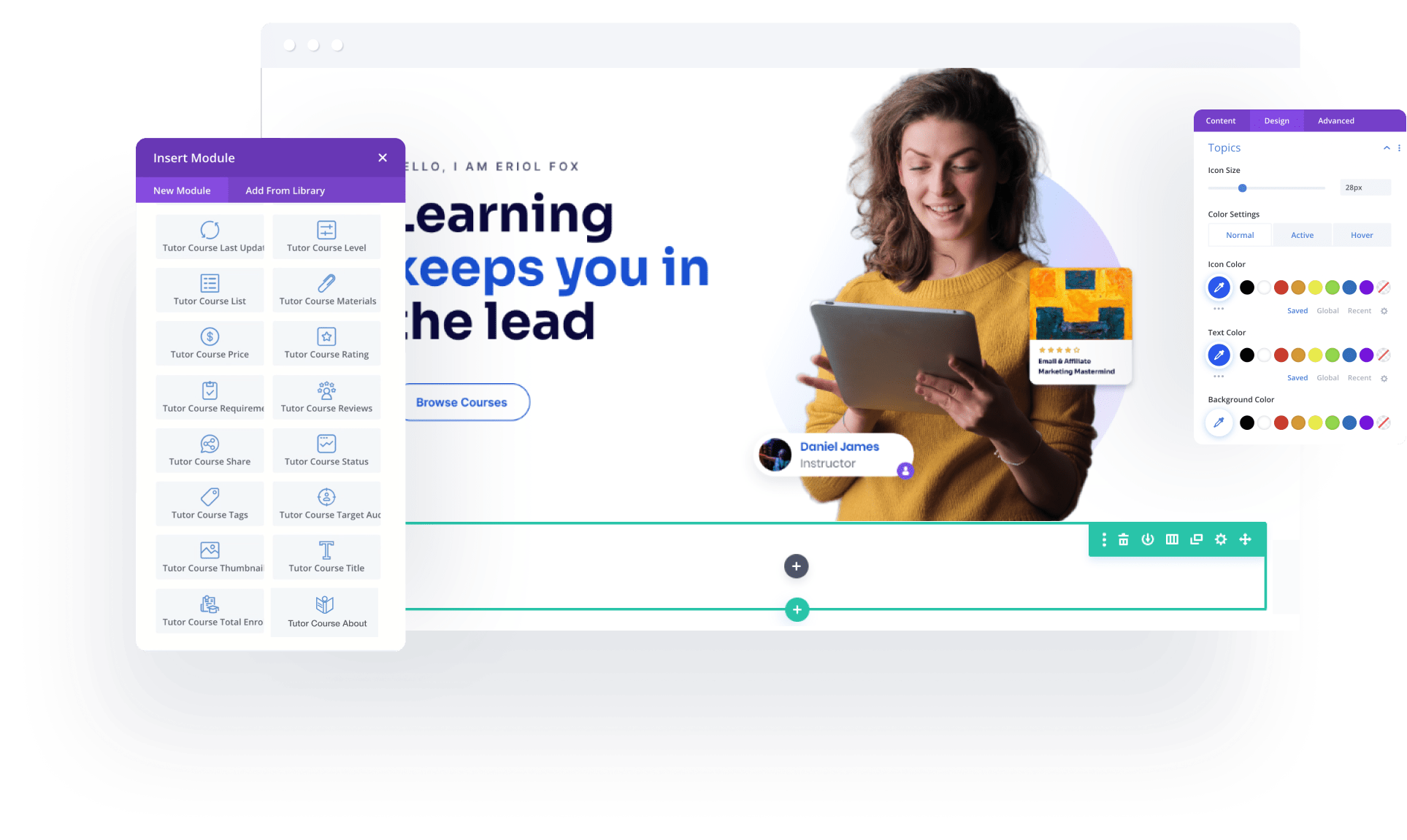This screenshot captures a section of a website and includes two open pop-up menus obscuring parts of the content. The image shows a gray navigation bar at the top with three white circles in the upper left corner. Below the bar, black text is partially visible on a white background. The visible portion of the text reads "Earning Eeps You In He Weed," which appears to be a truncated version of "Learning Keeps You In The Weed" due to the popup obscuring letters L, K, and T.

Prominently featured in the image is a photograph of a white woman with messy, hairspray-laden brunette hair. The woman appears to be making a surprised and delighted expression that seems exaggerated and somewhat condescending. She is dressed in an unattractive green sweater and is holding a large tablet, presumably tied to the context of the website, which is likely related to learning.